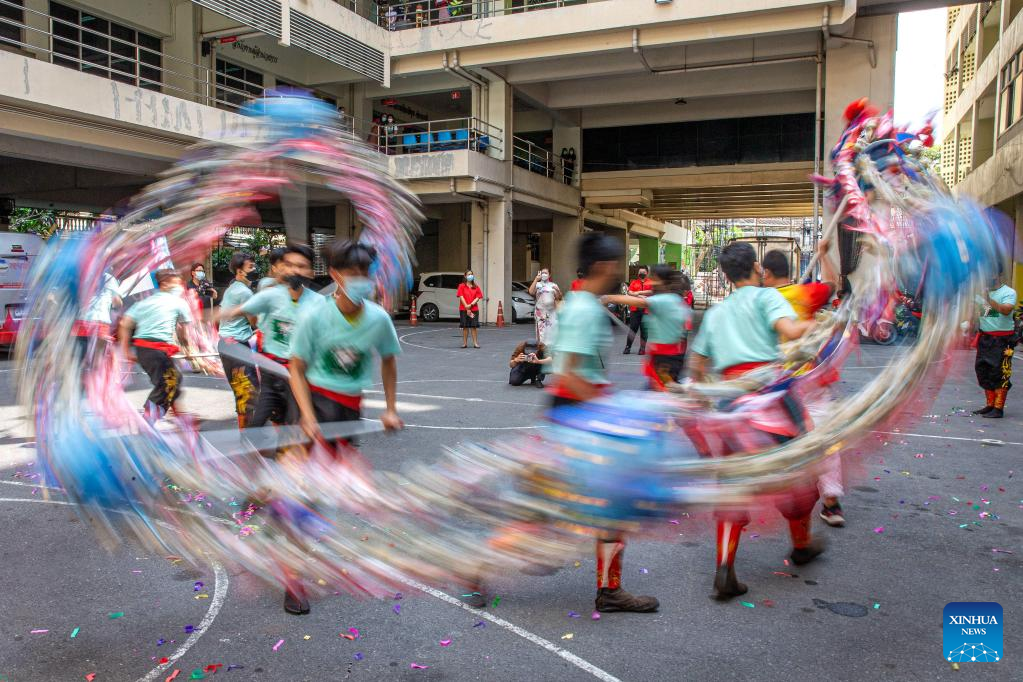This image captures a dynamic scene of children dancing in an alley, their movements creating a blur as they run around in a circle. They are all dressed alike in light blue shirts, black pants, and red socks, and they wave a colorful banner that is rendered indistinct due to the motion. This lively event takes place on what appears to be a blacktop or a basketball court, set within a wide-open space surrounded by buildings and parking spaces to the left. The backdrop features several adults, possibly parents or guardians, watching and taking photos. Notably, many in the crowd are wearing masks. A small detail in the bottom right corner of the image states "Xinhua News," suggesting that this scene is set in China. The well-lit setting, combined with the energetically blurred motion of the children, conveys an event filled with spirited activity and cultural significance.